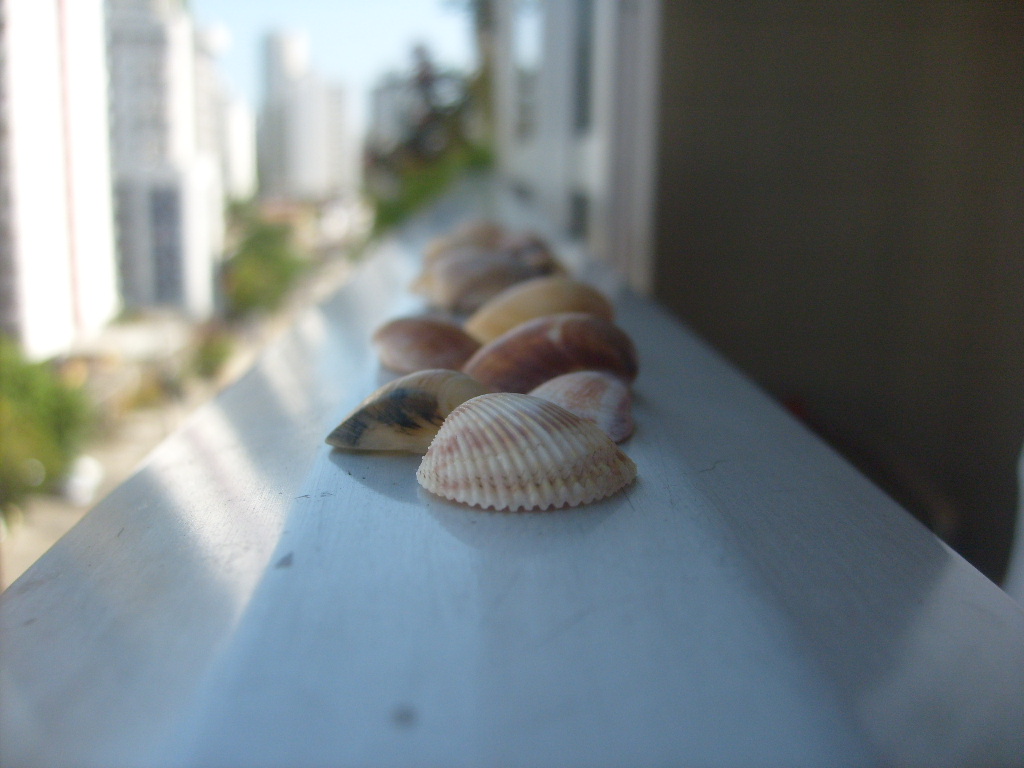This photograph captures a row of seashells meticulously arranged on a white banister outside a hotel room or an apartment balcony, against a backdrop of a bright sunny day with a clear blue sky. The seashells are lined up in a straight but alternating pattern, providing a visually appealing display. The shell closest to the viewer is a striking orange and white striped clam shell, followed by a brown and beige one. There are additional shells, varying in colors and types—some white with brown spots, others brownish with black, reddish, and yellowish—forming a sequence that converges into a blur as they stretch into the background. The right side of the image features a segment of a dark gray wall and windows, hinting at the building's exterior. In the blurred background on the left, green trees and urban elements suggest a metropolitan setting, potentially placing this balcony several floors above the ground. The meticulous focus on the seashells contrasts with the softer focus of the distant elements, creating a harmonious blend of detail and depth in the photograph.